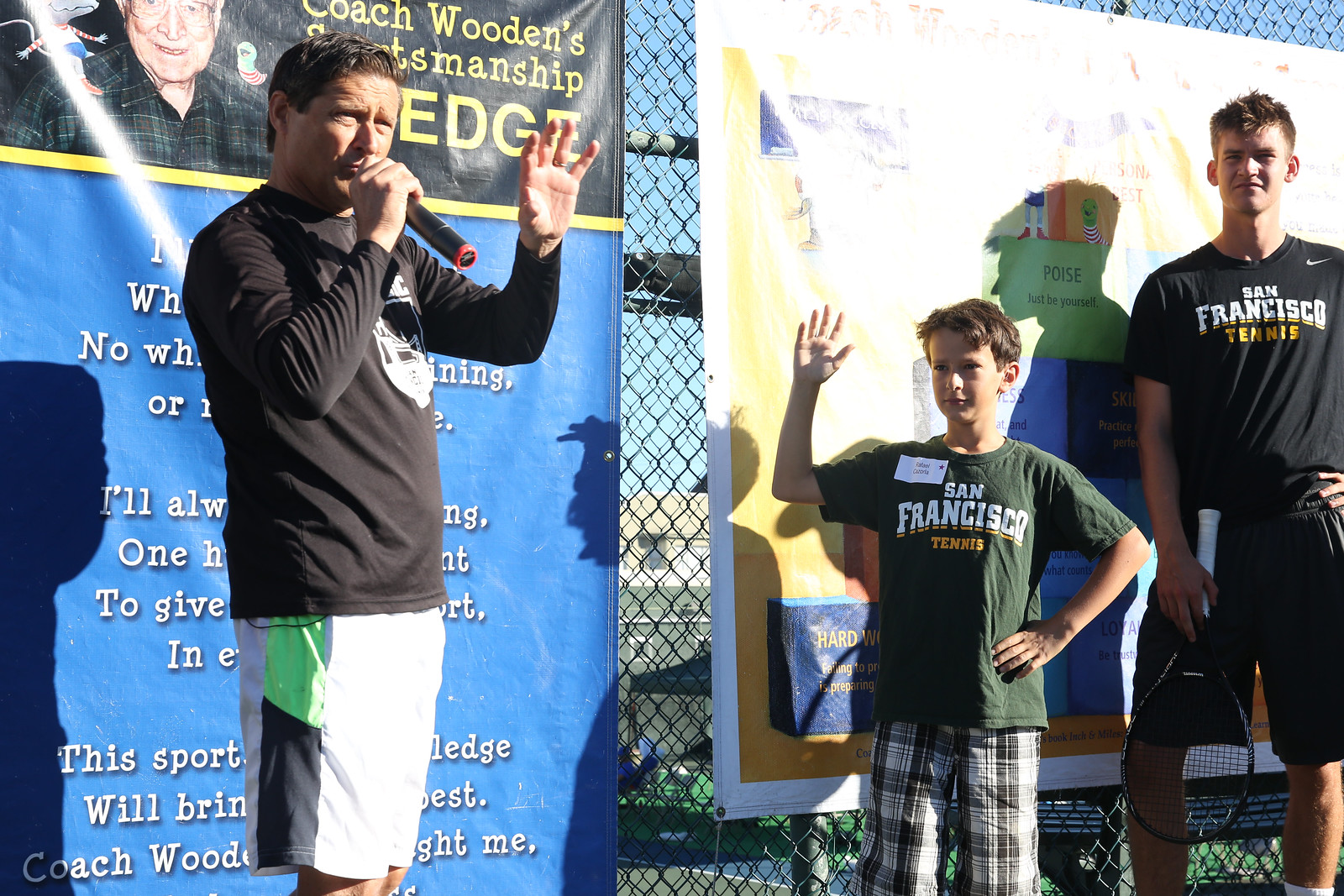In this vibrant outdoor scene, a rectangular photograph captures three figures against a chain-link fence adorned with welcoming posters. On the far left stands an adult male, dressed in a dark, informal long-sleeved t-shirt with a distinctive emblem on the front, and knee-length white shorts accented with green and black trim. He has short dark hair and is holding a wireless microphone to his mouth with his right hand. His left hand is raised, elbow bent at a 90-degree angle, as if engaging an unseen audience. 

To his right, slightly center-left in the image, is a young boy, likely around 10 years old, with short brown hair. He wears a dark gray or green t-shirt emblazoned with "San Francisco" in white lettering and "tennis" in gold or orange. A name tag is visible on the left side of his shirt. His right hand is raised with fingers splayed, and his left arm is akimbo, resting on his hip. He wears plaid shorts featuring shades of gray, black, and possibly yellow.

On the far right is a taller boy, appearing to be around 16 or 17 years old, and the tallest of the trio. Dressed in a similar t-shirt as the younger boy, his appears darker, possibly black, with identical white and orange lettering. He wears black shorts and stands with his right hand resting on his right thigh, while his left arm is mostly out of the frame, a hand visible on his left hip.

All the individuals appear Caucasian and cast strong shadows behind them, indicating a bright, sunny day. They stand in front of a chain-link fence adorned with promotional posters, one of which features the words “Coach Wooden’s Sportsmanship” alongside a picture of John Wooden and an inspiring quote against a blue backdrop. The second poster is more washed out by the sun, revealing a burst of multicolored text behind the group. 

Together, they present a vivid, dynamic image of a sunny day, perhaps at a sports event or community gathering.